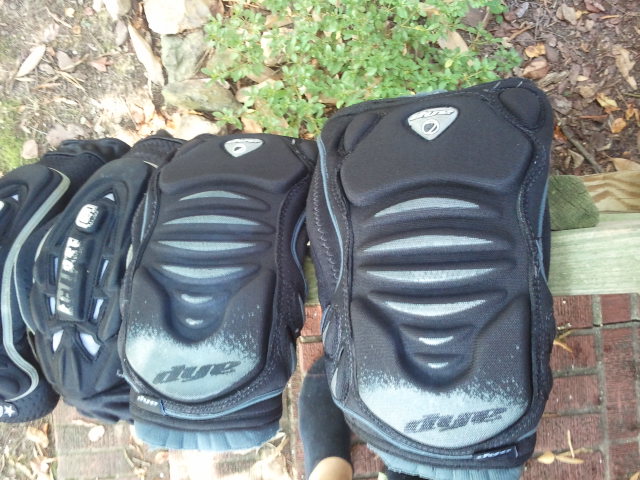The image features three pieces of black sports equipment, possibly boxing or sparring pads, bearing the brand name "DYE." The gear, which looks like it might be designed to protect the hands, knees, or elbows, is made of black plastic with foam padding. The scene is set outdoors, atop a red brick surface that appears to be part of a deck or stoop, with some green moss or a similar substance visible on the wood. A white person's foot, clad in a black sock, is partially visible on the left side of the image. In the background, other elements such as mulch, rocks, sticks, a small green bush, and some soil can be seen, adding to the detail of the natural outdoor setting. The photo has a generally bright yet gloomy ambiance and is taken from a top-down perspective, encompassing a square rectangular frame.